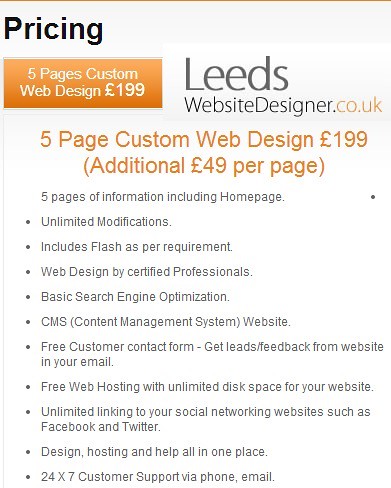**Advertisement for Web Design Services by LeedsWebsiteDesigner.co.uk**

In the top left corner, the word "Pricing" is prominently displayed in black. Underneath, an orange box announces the offer: "5 pages custom web design, £199." To the right, the company's name, "LeedsWebsiteDesigner.co.uk," is shown. Reiterated in the center, the offer "5-page custom web design, £199" is highlighted in orange text, with a note underneath stating "(additional £49 per page)."

The detailed packages include:
- **5 pages of information including the homepage**
- **Unlimited modifications**
- **Flash inclusion as per requirement**
- **Web design by certified professionals**
- **Basic search engine optimization (SEO)**
- **Content Management System (CMS)**
- **Free customer contact form**
- **Free web hosting with unlimited disk space**
- **Unlimited linking to social networking websites like Facebook and Twitter**
- **Design, hosting, and help all in one place**
- **24/7 customer support via phone and email**

This comprehensive service ensures that all your web design needs are met with professional quality and round-the-clock support.